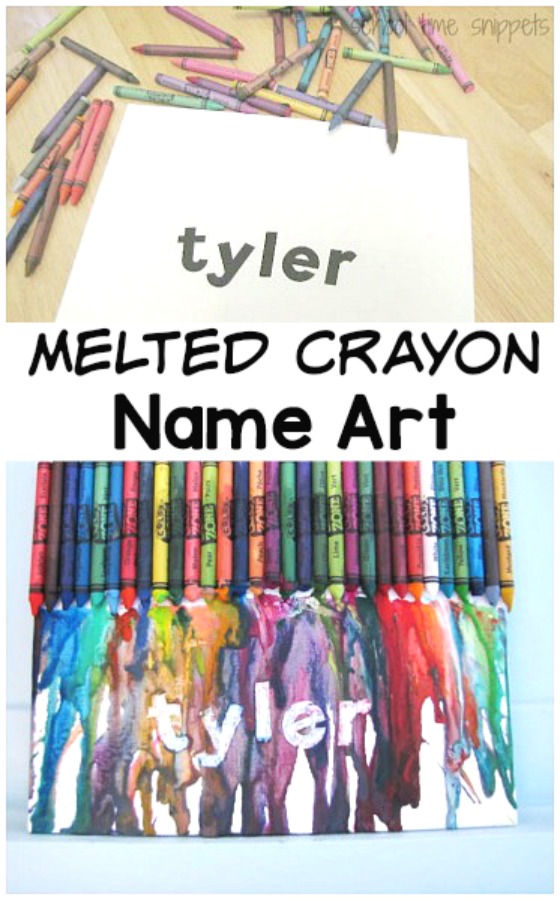The image presents a creative depiction of melted crayon name art, composed of distinct sections. In the top section, set against a light brown wooden floor, lies a white piece of paper with the name "Tyler" inscribed in block lettering. Various colored crayons are scattered around this paper, creating a vibrant frame. The middle section features a white background with the phrase "Melted Crayon Name Art" written in bold, black text. The bottom section showcases an artistic masterpiece: crayons arranged vertically, aligned side by side, their melted wax streaming down in vivid streaks onto a white sheet of paper, also bearing the name "Tyler." The overall composition illustrates the transformation of simple materials into a colorful, personalized piece of art.